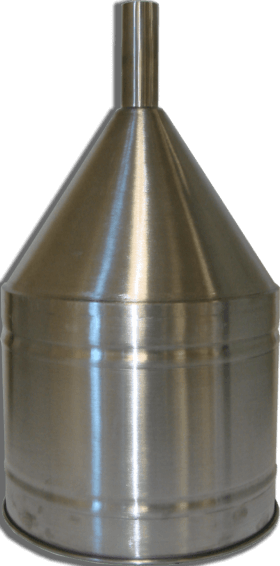The image displays a highly polished metallic hopper, characterized by a cylindrical base that transitions into a conical top ending in a pointed spout. The metal construction has a shiny, silver finish with a black trim around the bottom edge, and it reflects blue and white light. The hopper is the sole subject of the photograph, which is set against a plain, white background with no additional objects or text. Visible signs of age include a minor dent along the bottom rim, where the metal is soldered to the base. The overall setting is well-lit, enhancing the visibility and clarity of the detailed features of the metallic hopper.